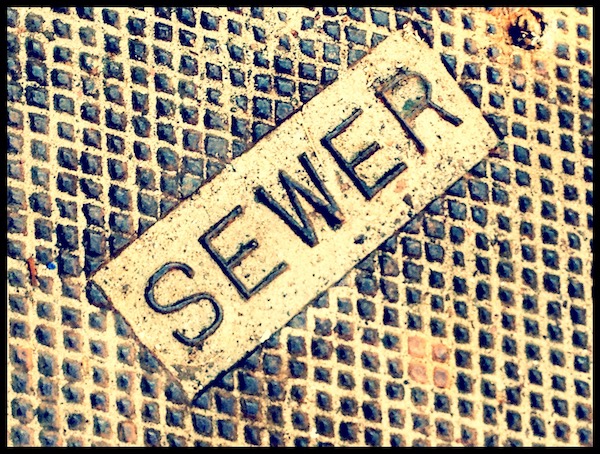This image features a close-up view of a worn-out sewer cover, typically seen in city streets or sidewalks across the United States. The metal cover prominently displays the word "SEWER" in large, uppercase black letters, slightly slanted and raised above a flat silver background. The cover is composed of a diamond plate design with raised, bumpy textures and several screws securing it in place. Predominantly black in color, the cover exhibits signs of heavy use and age, such as rust, stains, and areas where the paint has worn off, exposing the underlying metallic surface. The rust has transformed parts of the cover to a lighter yellowish hue, and the texture appears bumpy and uneven. Despite its aged and dirty appearance, the intricate details of the metalwork and its enduring presence are clearly visible in this close-up shot.